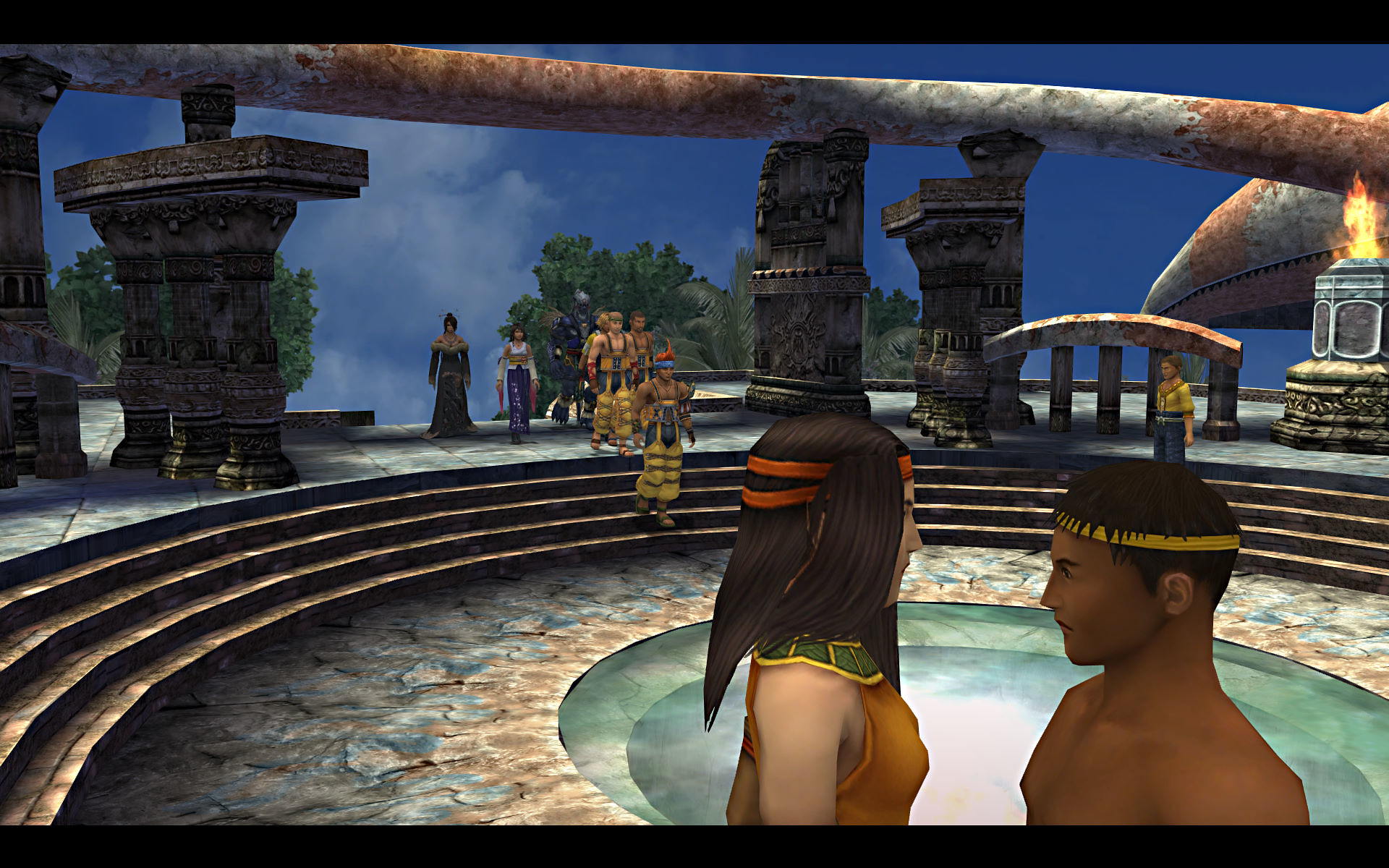In this computer-generated image from the video game Final Fantasy X, a detailed outdoor temple scene unfolds. Centrally placed towards the left, a group of characters gathers amidst ancient stone pillars that define the structure's grandeur. Just beneath these pillars, steps descend to a lower level where, in the bottom right-hand corner, a woman and a man face each other, perhaps engaged in a poignant moment.

The background of the scene features a bright blue sky adorned with very white, almost smoke-like clouds to the left. On the right, a flame dances atop a small pillar, emanating from a stone-like base, adding a touch of mystic ambiance. At the very bottom of the stone structure, a circular sphere is visible, perhaps a significant artifact within the game's narrative. The intricate details and evocative atmosphere encapsulate the fantasy adventure essence of Final Fantasy X.